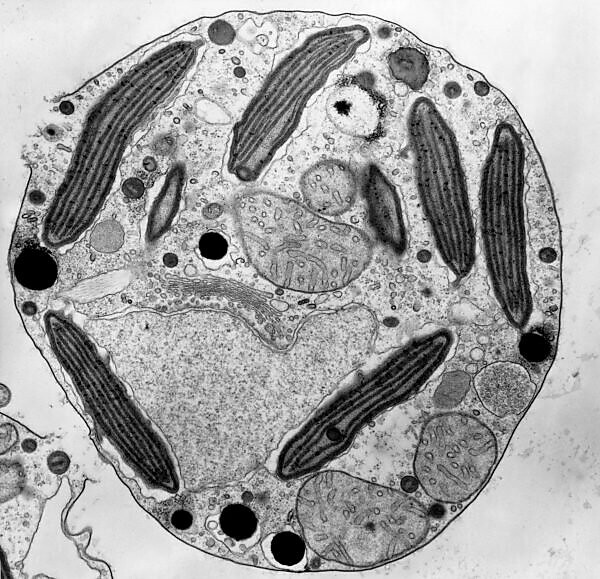The image displays a black and white microscopic slide, with the primary focus being a large circular cell. This cell features an assortment of internal components varying in shape, size, and shading. Dominating the cell's interior are several darker, elongated structures that resemble squiggly lines or "pickle-like worms," interspersed with lighter, larger circular shapes that have walls around them dotted with finer details. These elements are set against a grainy or "gravelly" textured background within the cell, contributing to its complex appearance. The cell is encapsulated by a distinct black outline, contrasting starkly with the plain white background outside. In the lower left corner, a separate shape is emerging, adding another layer of interest to the image.